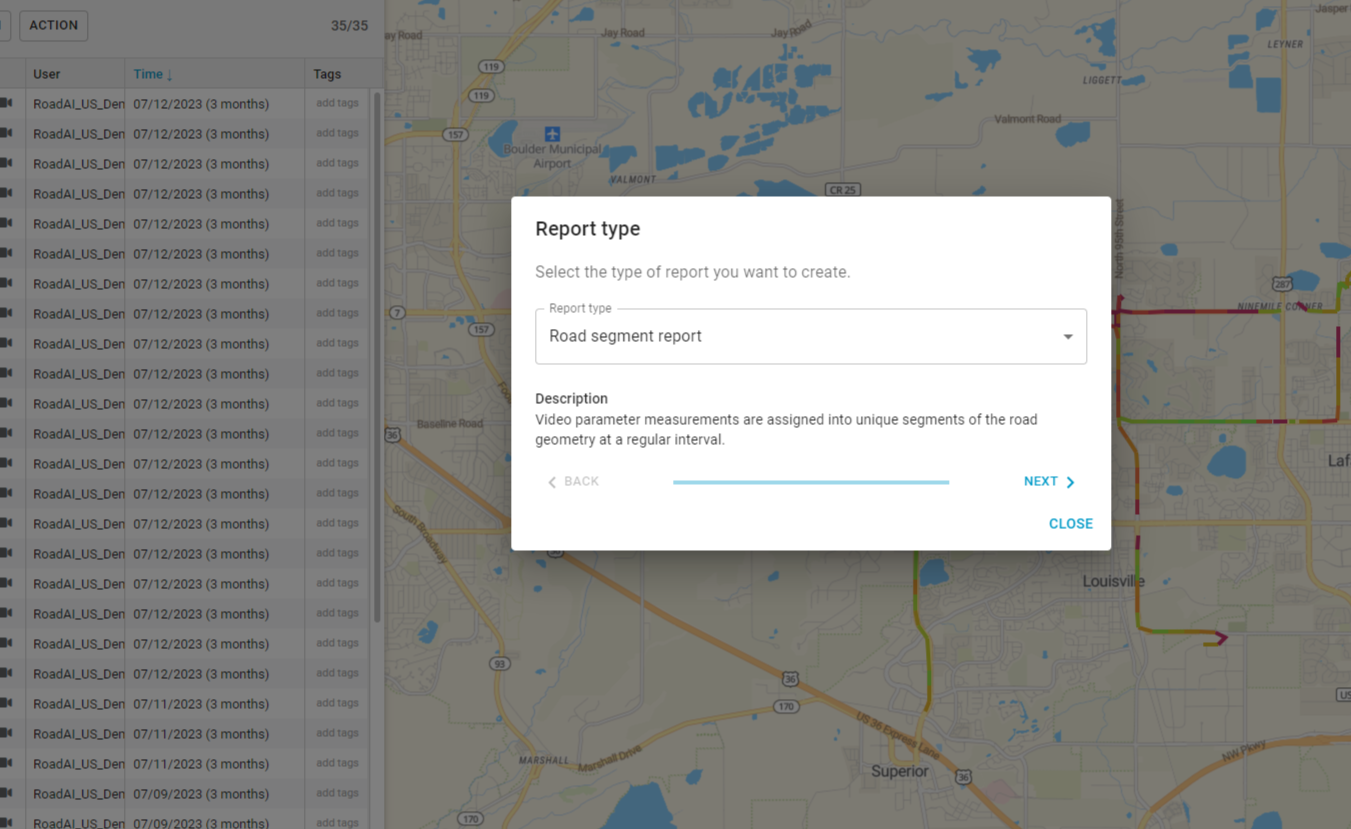The image depicts a Google Maps screenshot or a similar mapping program with a gray tint rendering the text barely legible. The map displays a terrain populated with numerous small lakes or ponds. A section of the map indicated in red signifies heavy traffic congestion, with the congestion feature activated. On the left side of the image, there is a box divided into three columns labeled 'User,' 'Time,' and 'Tags.' Each entry within this box includes a filename and is dated 07-12-2023, suggesting a date three months in the future. Additionally, a middle overlay box titled "Report Type" prompts the user to select the type of report they wish to create. This box includes a dropdown menu with an option for a 'Road Segment Report' and offers 'Next' and 'Close' buttons at the bottom.